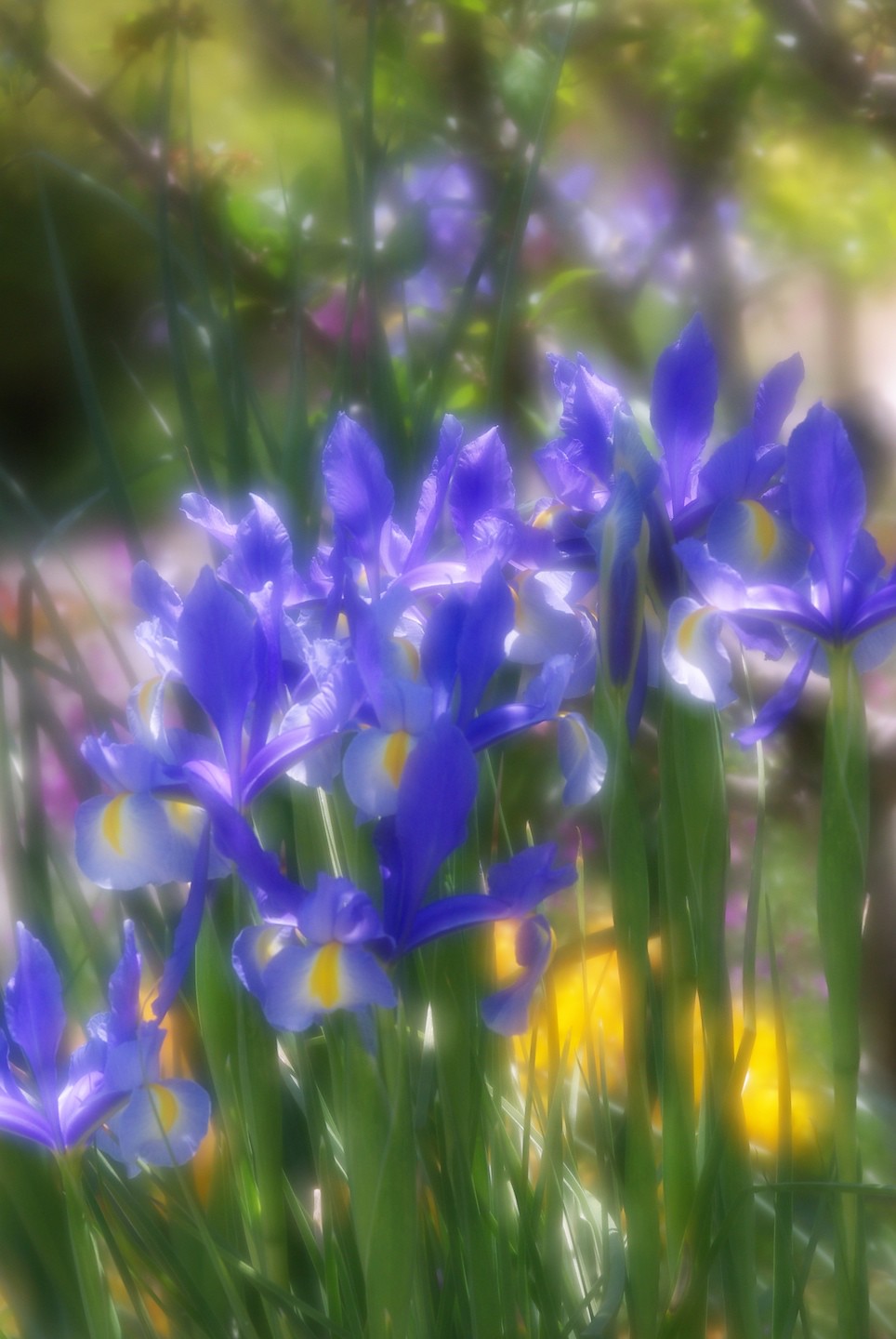This close-up image captures a small cluster of six slender, green-stalked Dutch blue irises with vivid, royal blue petals reaching upward. Each petal is accentuated by a delicate yellow section outlined in white, giving a striking contrast. The bright sunlight illuminates the scene, filtering through and highlighting the intricate features of the irises' petals while leaving the background in a dreamy blur. In the background, various shades of green from stems and leaves, along with faint hints of purple and possible yellow flowers, create a lush, soft-focus backdrop that further emphasizes the sharp beauty of the irises in the foreground.